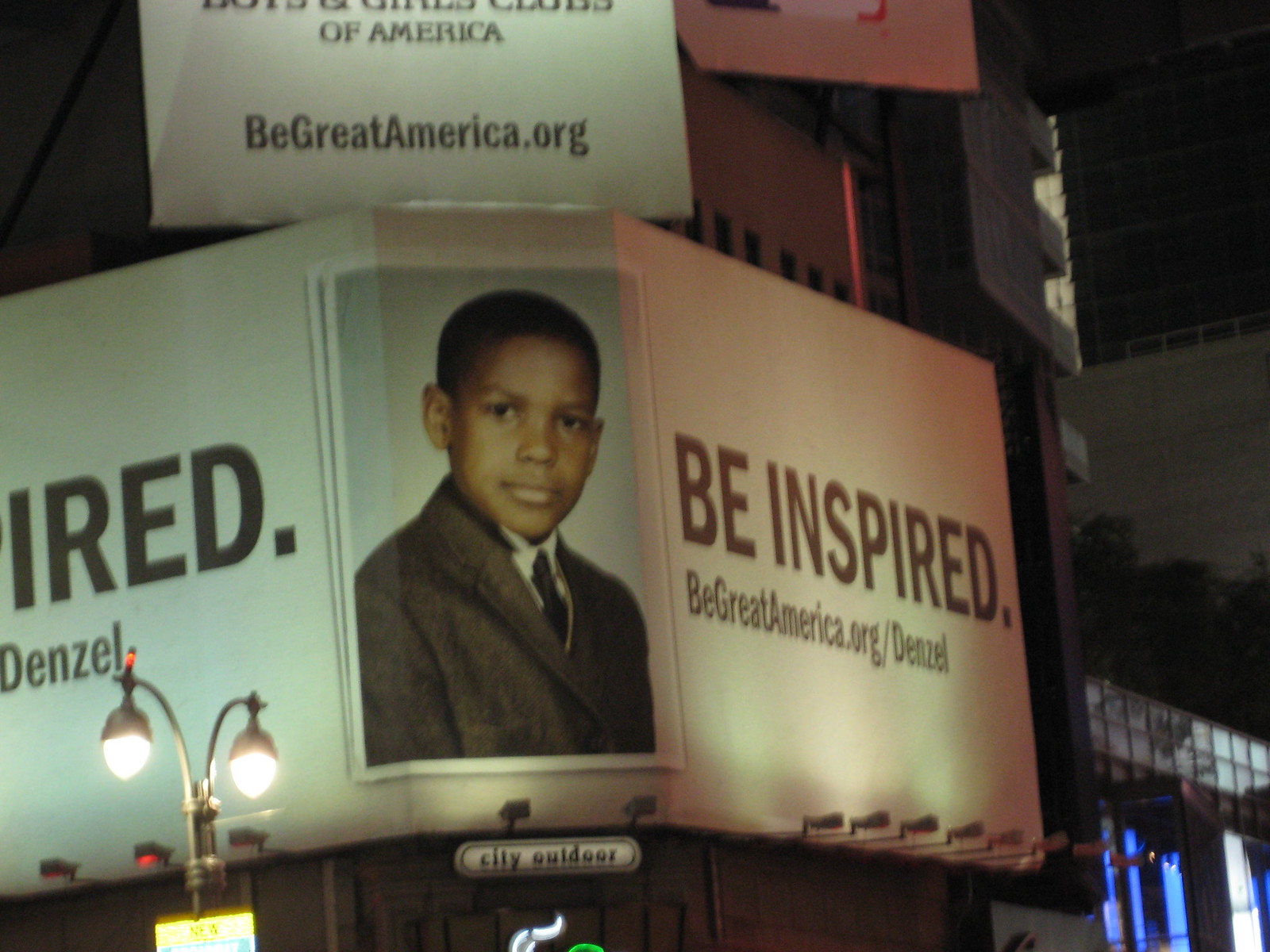A nighttime outdoor photograph, slightly blurred, captures the side of a building illuminated by street lamps near the bottom of the frame. Dominating the image is a large advertisement. The central feature of the advertisement is a photo of a young Black boy dressed in a smart brown jacket and tie, bearing a serious expression. The text accompanying the photo reads, "BeInspired. BeGreatAmerica.org," urging onlookers to visit the website, BeGreatAmerica.org.